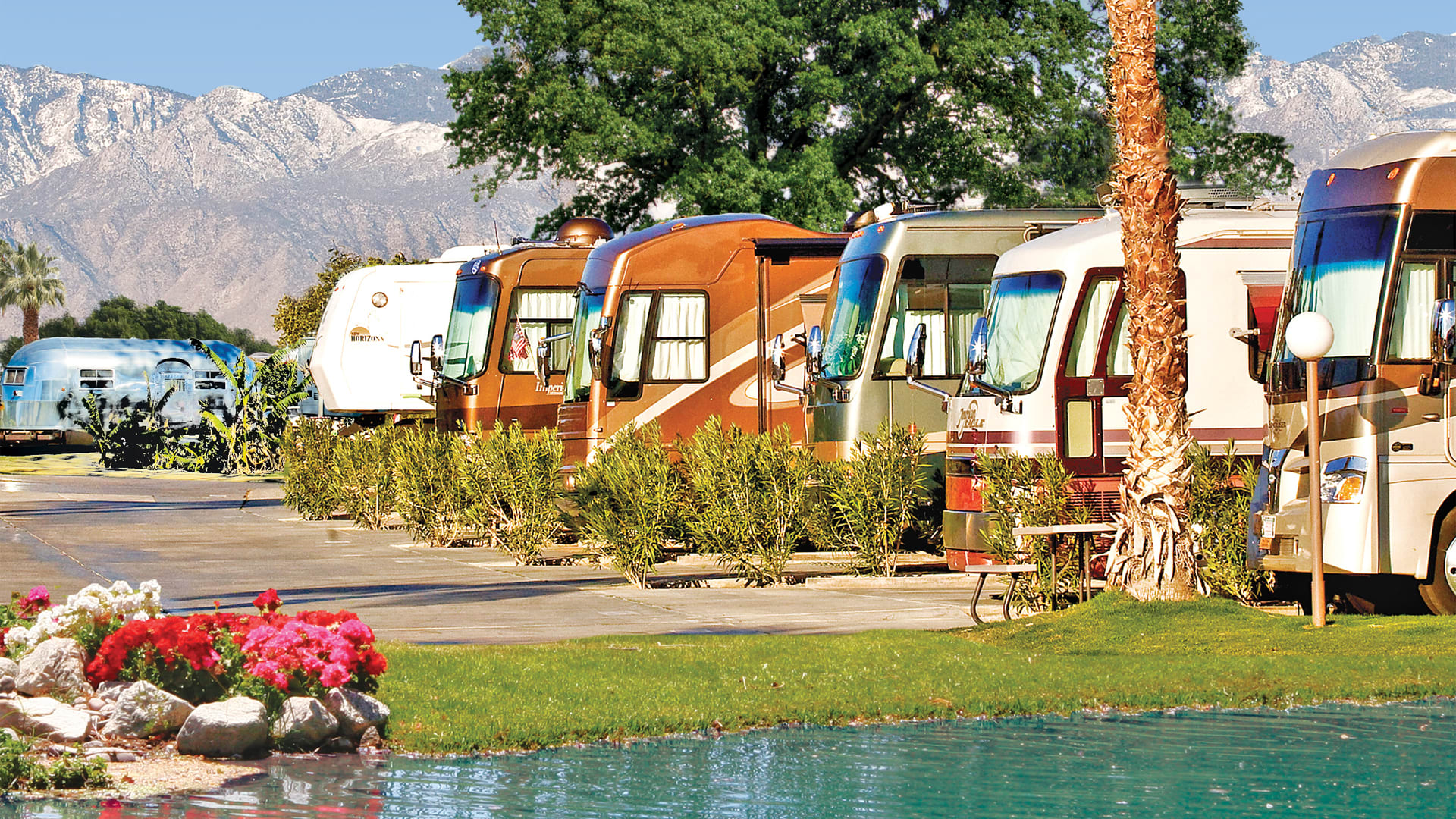The image depicts a slightly upscale trailer park or RV park nestled against a scenic backdrop. There are six trailers and RVs, of which three are white, one gray, two wooden orange, and one light blue. The park features a diversity of vegetation, including a large, skinny-trunked tree with green canopy located near the first trailer, as well as various smaller plants and scrub brushes lining the RVs. In the foreground, there is a picturesque pond edged with rocks and adorned with vibrant flowers in red, white, and pink hues, as well as patches of green grass. A neat sidewalk runs through the park, providing a walkway for residents. The background boasts a majestic mountain range extending across the image, complementing the lush greenery and a clear blue sky, enhancing the serene and welcoming environment of the park.